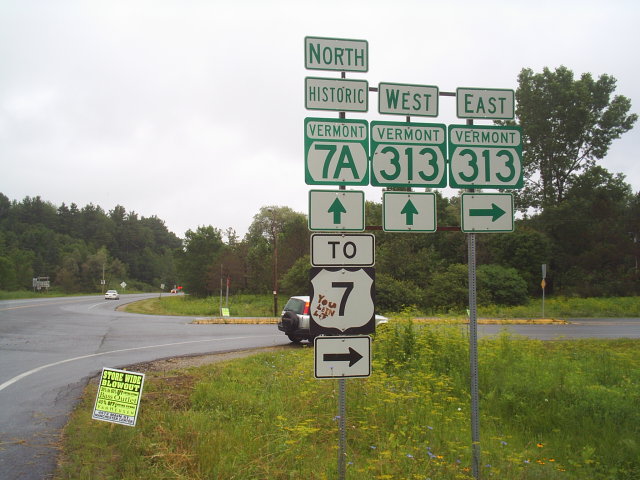This photograph captures a quaint rural intersection on an overcast day, with a backdrop of lush green deciduous trees. The sky is heavily clouded, casting a soft light across the scene. A blacktop road curves to the right while continuing straight ahead, with a white car parked at the bend and another further down the straight stretch.

The focal point of the image is a cluster of directional signs situated at the intersection, each with a distinctive white background, green edging, and green lettering. The signs guide travelers in various directions:

- At the top of the first sign, the word "NORTH" is prominently displayed in capital letters, followed by the word "HISTORIC" and an arrow pointing right. Below it, "Vermont 7A" is written with an arrow pointing straight. Lastly, a sign with "TO" in black letters is paired with a shield bearing the number "7" and an arrow pointing right.

- The second sign directs travelers "WEST" toward "Vermont 313" with a green arrow indicating a straight path ahead.

- The third sign points to the "EAST," also for "Vermont 313," with a green arrow directing to the right.

Nestled among the directional signs is a small, vibrant yellow sign stuck into the ground, announcing a "Storewide Blowout," though the finer details are unreadable. This scene, with its blend of functional road signs and the hint of local commerce, offers a charming snapshot of rural Vermont life.